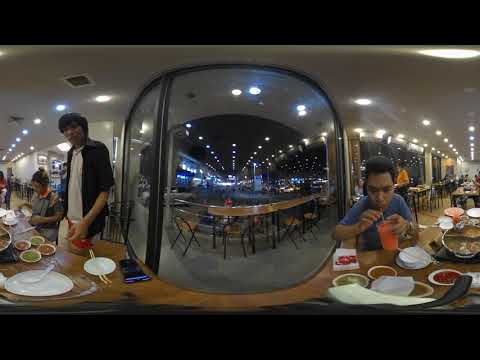In this panoramic photograph taken inside a bustling restaurant, the scene is divided into various focal points that capture the lively atmosphere. On the left side, a man with dark hair, dressed in a blue shirt, is seated at a table filled with an assortment of dishes, including what appear to be sauces or dips. He is drinking an orange-colored liquid through a straw from a clear cup. Moving towards the center, a large, rounded square window reveals the outdoor setting with empty tables and chairs, a row of distant lights, and a glimpse of the cityscape. The right side of the image features a man standing in front of a table. He is wearing a white t-shirt layered under an unbuttoned black shirt. Next to him, a short person stands close by. Their table is also adorned with dishes and chopsticks. Above, the ceiling is lined with vents and a row of lights, adding to the ambiance. A woman stands to the left of the man in the black shirt. The overall composition of the image creates a vivid, almost surreal sense of being both inside the restaurant and peering into its outdoor surroundings simultaneously.